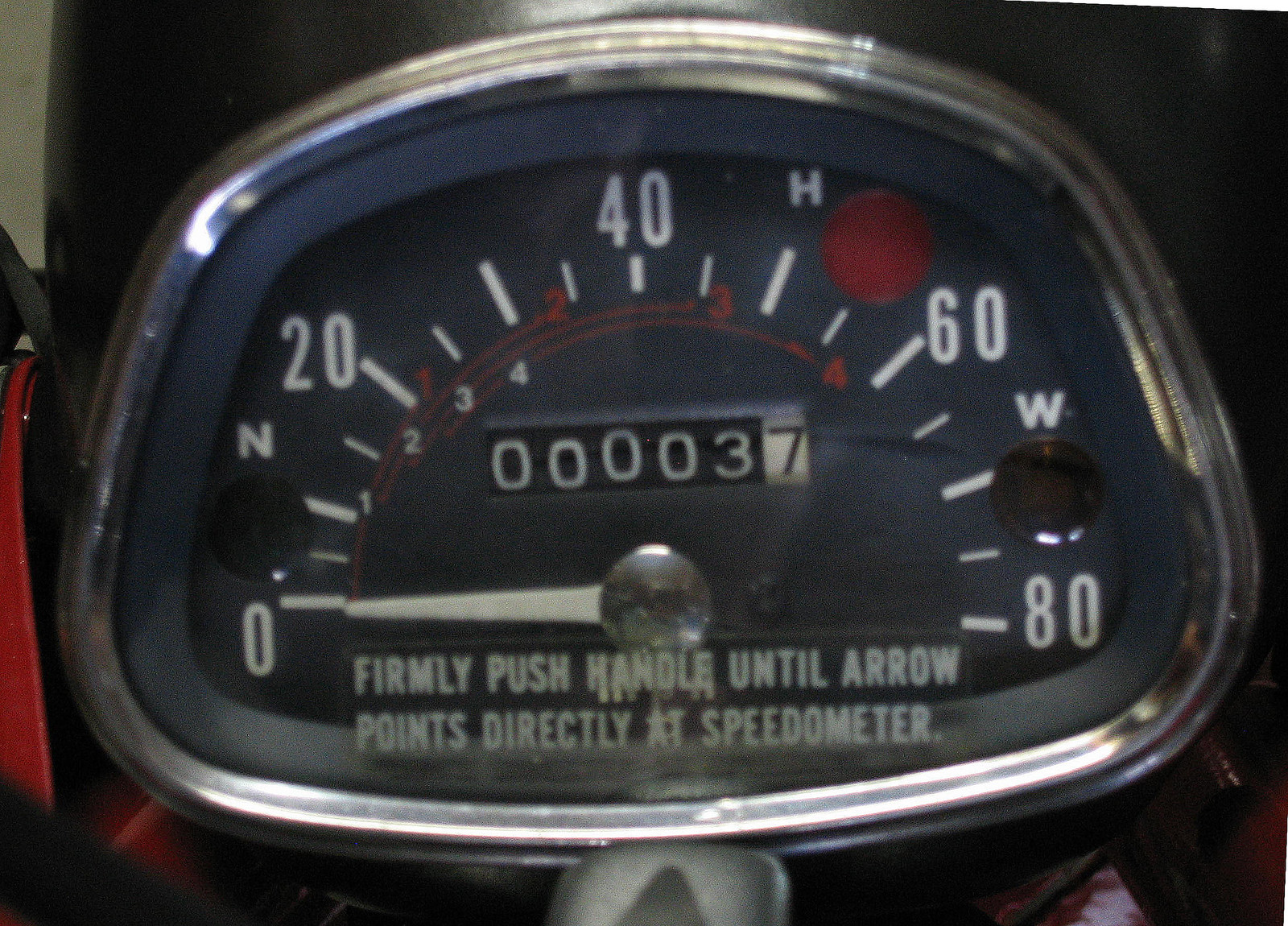Close-up photograph of a vintage speedometer set against a black background. The speedometer has a unique, almost mushroom-shaped design with a thick, silver metallic exterior frame. Nested within this frame is a smaller black border, inside which lies the main face of the speedometer, also black in color. The speedometer scale starts from 0 and goes up to 80, with white numerals marking every 20 units (0, 20, 40, 60, 80). Smaller white numbers are positioned between the 10 and 30 marks, while tiny red numbers are placed between the 20 and 60 marks. Between the 40 and 60 on the arc, there is a large red dot adjacent to an "H". Between the 60 and 80 marks, a black dot with a "W" above it is visible. The speedometer features a glass cover with the instruction "firmly press handle until arrow points directly at speedometer" inscribed on it. The dial is silver and round, with a white pointer arm emanating from its center. The overall craftsmanship and intricate details suggest a precise, well-engineered device likely used in a mechanical or automotive context.